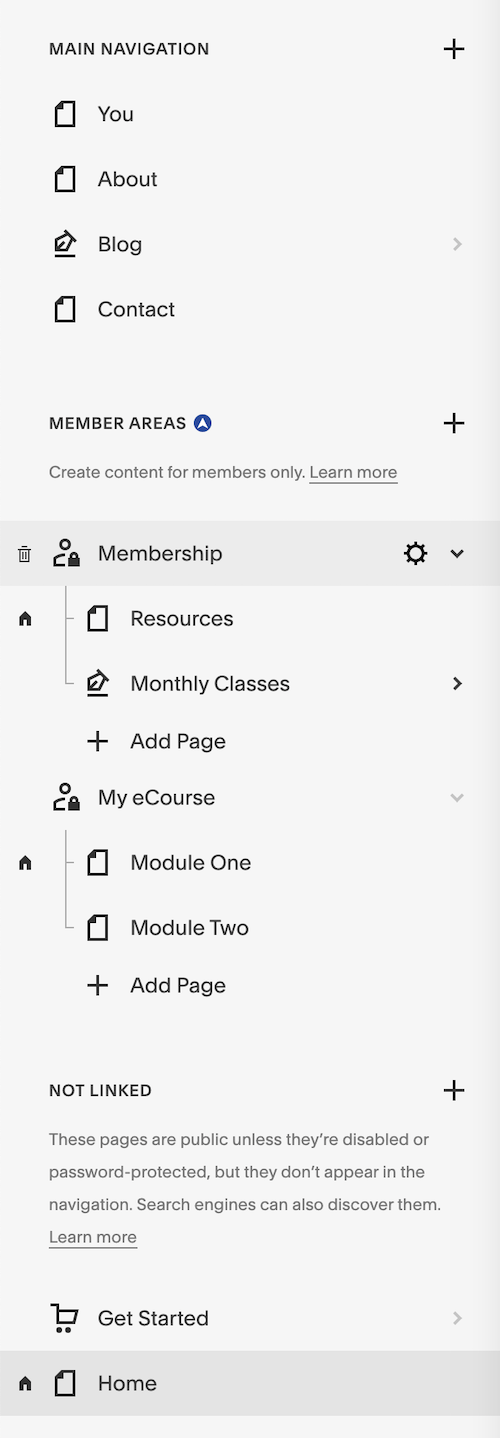The image showcases a menu interface set against a gray-colored background. At the top, there is a section labeled "Main Navigation," which includes a plus sign to the right and various document icons for different sections: "You," "About," "Blog," and "Contact." Below this, there is a "Members Area" section featuring a blue circle with an upward arrow next to a plus sign, accompanied by the text, "Create Content for Members Only," and a "Learn More" link.

Additionally, there is a "Membership" button, bordered in a slightly darker gray than the rest of the menu, adjacent to a cogwheel icon with a drop-down options menu. This drop-down menu includes entries such as "Resources," "Monthly Classes," "Add Page," "My E-Course," "Module 1," "Module 2," and another "Add Page."

Further down, a section labeled "Not Linked" contains a plus sign on the right and explains that these pages are public unless disabled or password-protected. It notes that unlinked pages do not appear in navigation but can be discovered by search engines, with links to "Learn More" and "Get Started."

Finally, the "Home" option is highlighted with a gray border, similar to the "Membership" option, indicating it is part of the main menu navigation.